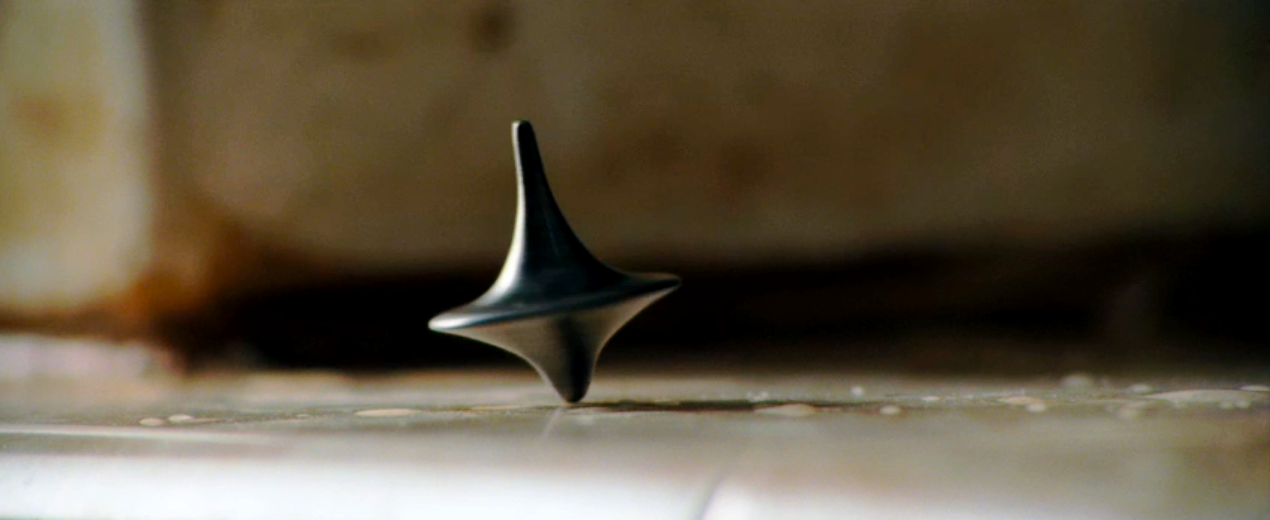This image captures a close-up, ground-level view of a dark, metallic spinning top, which appears to be in mid-motion, balanced upright on its point, and tilted slightly to the left. The top is dark greenish-black or dark gray and resembles a dreidel or a simple spinning toy made of metal. Light from the left side reflects off the top, casting a subtle shadow on the floor. 

The floor, likely made of white or off-white ceramic tiles, shows some evidence of wear and features water droplets and possible grout lines, indicating a somewhat aged and possibly dirty surface. In the blurred background, the scene is divided into distinct sections: a dark strip through the middle, a tan or cream-colored area with brown and orange residue or spotting above it, and a discolored, possibly tiled or stone wall at the bottom. This wall features irregular patterns of white, brown, and tan, with a black streak near the base, adding to the overall gritty and aged aesthetic of the setting. The background and floor contribute to an impression of an old, perhaps neglected, environment.